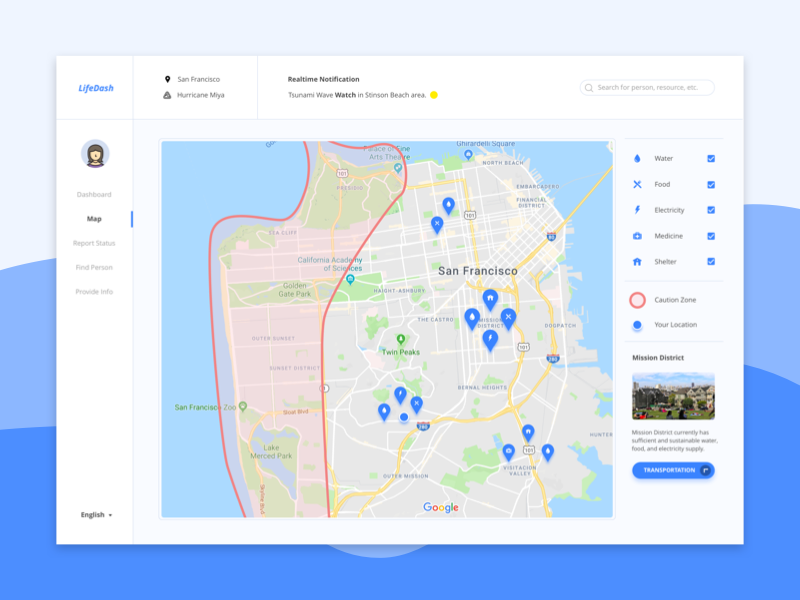Detailed Caption: 

The image showcases an app or website named "LiveDash," designed for tracking caution zones and dangerous areas during a disaster. The interface features a clean white main page set against a multicolored background with gradients of light blue and darker blue hues.

In the top left corner of the screen, the "LiveDash" logo is prominently displayed, followed by the location marker, "San Francisco," and the disaster label, "Hurricane Mia." Directly to the right, a real-time notification alerts users about a "tsunami wave watch in Stinson Beach area." Near the top right corner, a search bar is available for user input.

On the left-side menu, a profile icon is positioned at the top, followed by navigational options including "Dashboard," "Map," "Reports," "Status," and "Find Person." The "Map" option is selected, leading to a large map of San Francisco dominating the center of the screen. The map, embedded with multiple pins and a prominent red outline around a caution zone, is visually informative.

To the right of the map, there is a detailed legend and information panel. This panel lists various icons and their respective meanings: water, food, electricity, medicine, and shelter. These icons are scattered across the map, indicating resource locations throughout San Francisco. A red circle icon denotes the caution zone, while a small blue dot indicates the current location of the user.

Beneath the legend, a suggestion highlights "Mission District" as a reliable support area, with a detailed description stating, "Mission District currently has sufficient and sustainable water, food, and electricity supply." Finally, a prominent blue "Transportation" button offers users guidance on how to reach the Mission District, providing a practical solution during the disaster.

This comprehensive setup ensures users are well-informed and can find necessary resources and safe zones effectively.